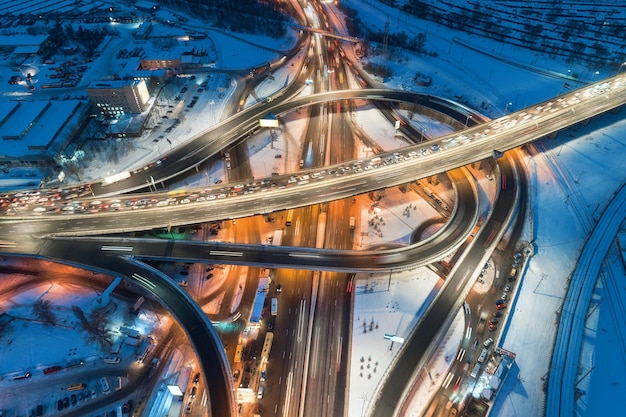This is an intricate aerial photograph of a snowy freeway interchange taken during an evening in a cold, winter cityscape. The image captures a complex network of freeways, roads, and off-ramps adorned with streetlights that illuminate the scene. The image features a prominent vertical freeway stretching from the bottom center to the top center, intersected by a curving horizontal freeway that runs from the left to the top right of the frame. The interchange is intricately designed with connecting roads arching and curving around each other, creating a labyrinth of pathways under and above one another.

The snow-covered ground casts a dark blue hue in each corner of the frame, further accentuating the winter setting. Traffic congestion is evident, with blurred lights of cars present on the closer side of the horizontal freeway and the top part of the vertical freeway, while vehicles on the far side of the horizontal freeway are at a standstill, bumper to bumper. A single beige building in the top left quadrant, accompanied by a parking lot dotted with small black cars, stands out as a notable landmark. The distant view includes trees and possibly residential areas, with some buildings showing lights, adding to the sense of a bustling urban environment enveloped in the serenity of a snowy night.